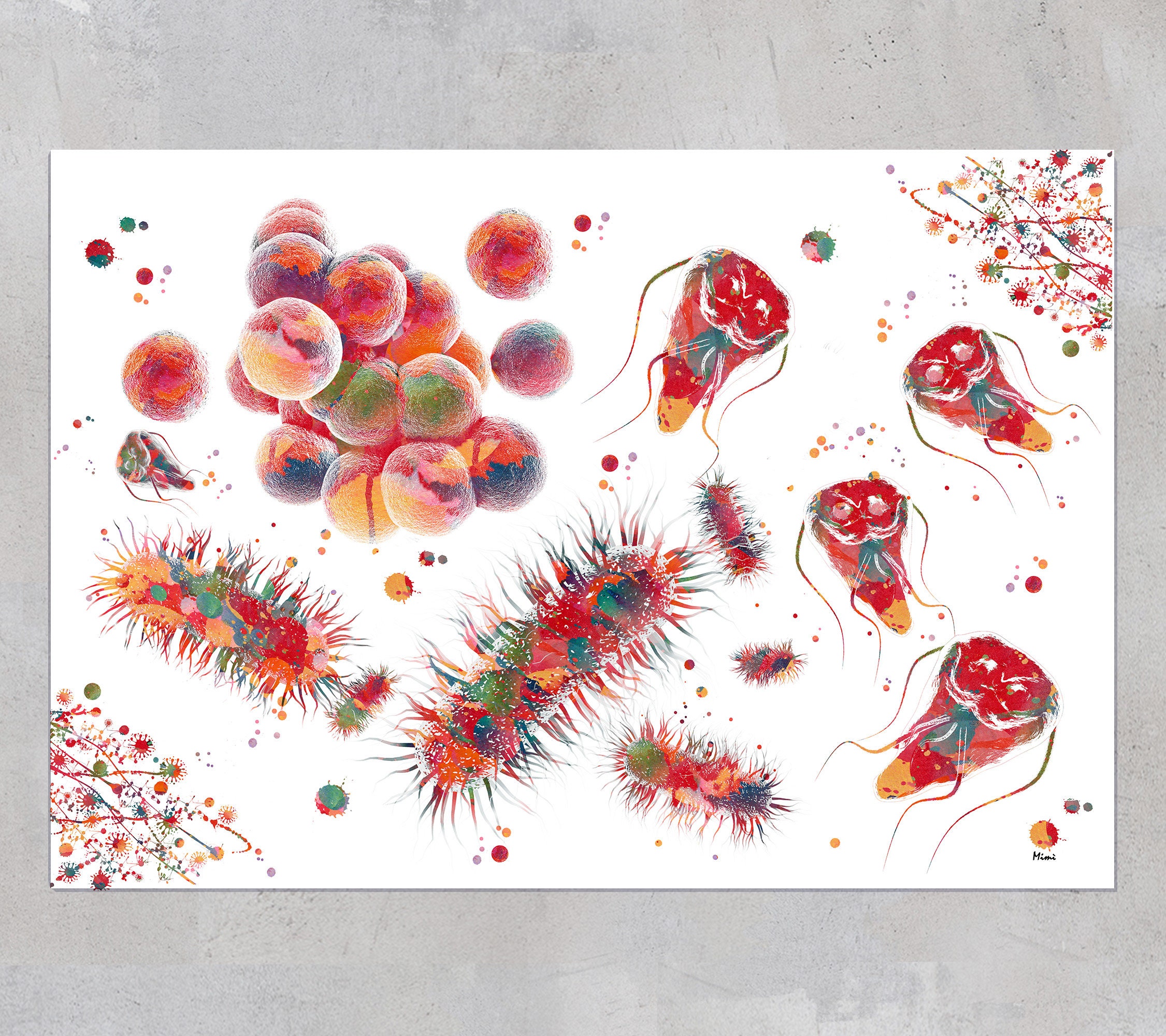The image features a whiteboard with a captivating and intricate array of colorful, hand-drawn objects. Predominantly, there are circles of various sizes and colors, including reds, greens, and blues, scattered across the board, giving it a vibrant, chaotic appearance. Among these circles, some are clustered together reminiscent of red blood cells. Additionally, there are peculiar, caterpillar-like figures with hairy edges, adding a textural element to the image, and these too are filled with an array of lively colors. Moreover, the illustration includes bug-like shapes adorned with long strings or appendages emanating from them, further enhancing the biological motif. Notably, the top right and bottom left corners feature smaller, detailed designs, populated with tiny circles and intricate lines that also burst with color. Throughout the whiteboard, one can spot random smaller circles and tiny undecipherable letters, all set against a light gray background, giving the scene a playful, microscopic feel.